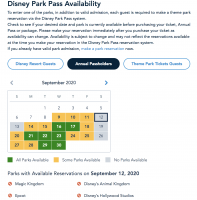A screenshot showcasing Disney Park Pass availability is set against a white background. The image includes a calendar for September 2000, navigable via a gray left arrow and a blue right arrow. The calendar is structured with dates ranging from the 1st, aligning under Tuesday, to the 30th, which falls under Wednesday. Specific dates on the calendar are color-coded: 

- Dates 9th, 10th, and 11th are marked in yellow.
- Dates 14th, 15th, 18th, 20th, 24th, 25th, 27th, and 28th are also yellow.
- Dates 12th, 13th, 19th, and 26th are colored gray.
- Dates 16th, 17th, 21st, 22nd, 23rd, 29th, and 30th are indicated in green.
  
A legend at the bottom of the screenshot explains the meaning of each color: green, yellow, and gray, which likely represent different levels of park pass availability.